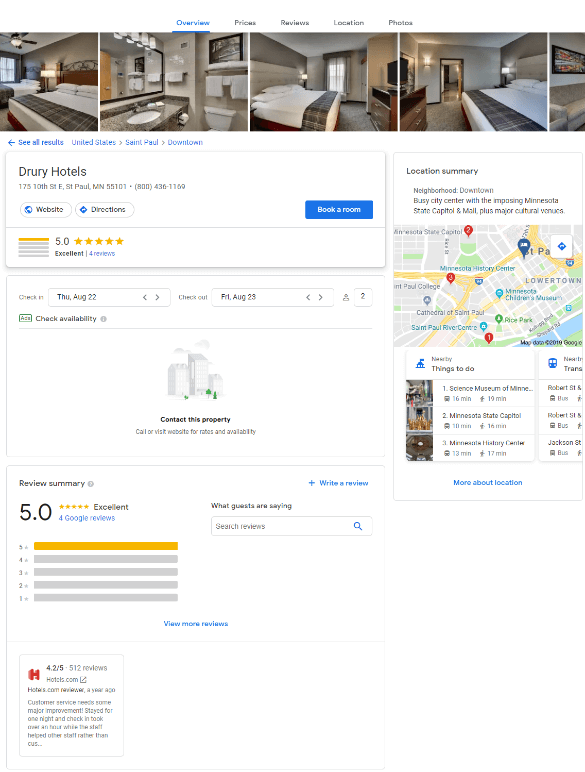Screenshot of Google Page for Hotel Listings

The screenshot displays a Google search results page focused on hotel listings, specifically for Drury Hotels in St. Paul, Minnesota. At the top of the page, there are five tabs labeled: Overview, Photos, Reviews, Location, and Photos.

The top section features a row of photographs depicting a hotel room. Below the images is a breadcrumb trail guiding through “See all results,” “United States,” “St. Paul,” and “downtown."

In the first chart, which is rectangular with a white background, the title "Drury Hotels" is displayed alongside its address in St. Paul, Minnesota, and the phone number: 800-436-1169. Two tags, "Website" and "Directions," are included. On the far right end, there is a blue “Book a Room” button. The hotel boasts a five-star rating from four reviews.

Beneath this, a wider chart details the check-in and check-out dates—August 22nd and August 23rd, respectively—with “Check availability” text under the check-in date. In the middle section, it says “Contact this property.”

The subsequent chart highlights a review summary with another five-star rating from four Google reviews. Adjacent to the rating section is a segment titled "What guests are saying," accompanied by a search bar for the review page. A blue link in the top right corner invites users to “Write a review,” while a smaller blue text in the center says “View more reviews.” In the bottom left corner of this section, a box shows a review from Hotels.com, indicating a rating of 4.2 out of 5 stars from 512 reviews.

The final chart, located on the far right, features a map with a caption "Location Summary" above it. Below the map, it lists nearby attractions such as the Science Museum of Minnesota, the Minnesota State Capitol, and the Minnesota History Center.